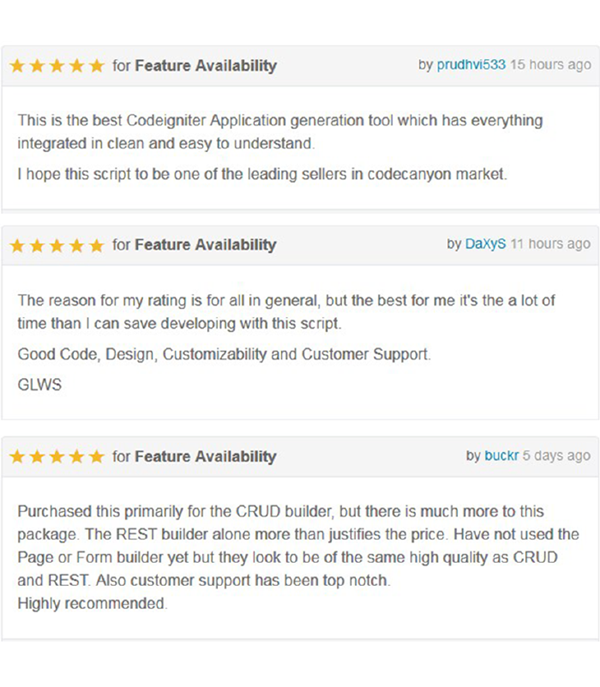This image presents a series of user reviews in a comment-style format, each enclosed in distinct boxes. The reviews are visually structured with a gray header section followed by a white text area. The reviews, all rated 5 stars for feature availability, provide comprehensive insights into a CodeIgniter application generation tool.

1. **Review by Prudhivi533 (15 hours ago):**
   - **Rating:** 5 stars for feature availability
   - **Review Content:** Prudhivi533 describes the tool as one of the best for CodeIgniter application generation, highlighting its integrated features, cleanliness, and user-friendly interface. They express optimism about the script becoming a leading seller in the CodeCanyon market.

2. **Review by DAXYS (11 hours ago):**
   - **Rating:** 5 stars for feature availability
   - **Review Content:** DAXYS praises the tool for its time-saving capabilities, good code quality, design, customizability, and customer support. They indicate that these qualities are the reason behind their high rating.

3. **Review by BuckR (5 days ago):**
   - **Rating:** 5 stars for feature availability
   - **Review Content:** BuckR notes utilizing the tool primarily for its CRUD builder but acknowledges the package contains much more. They specifically applaud the REST builder, suggesting it alone justifies the price. Although they have not yet used the page or form builder, they anticipate it to be of similar high quality and commend the top-notch customer support, concluding with a strong recommendation.

The overall consensus from these reviews is that the CodeIgniter application generation tool excels in feature availability, ease of use, and customer support.